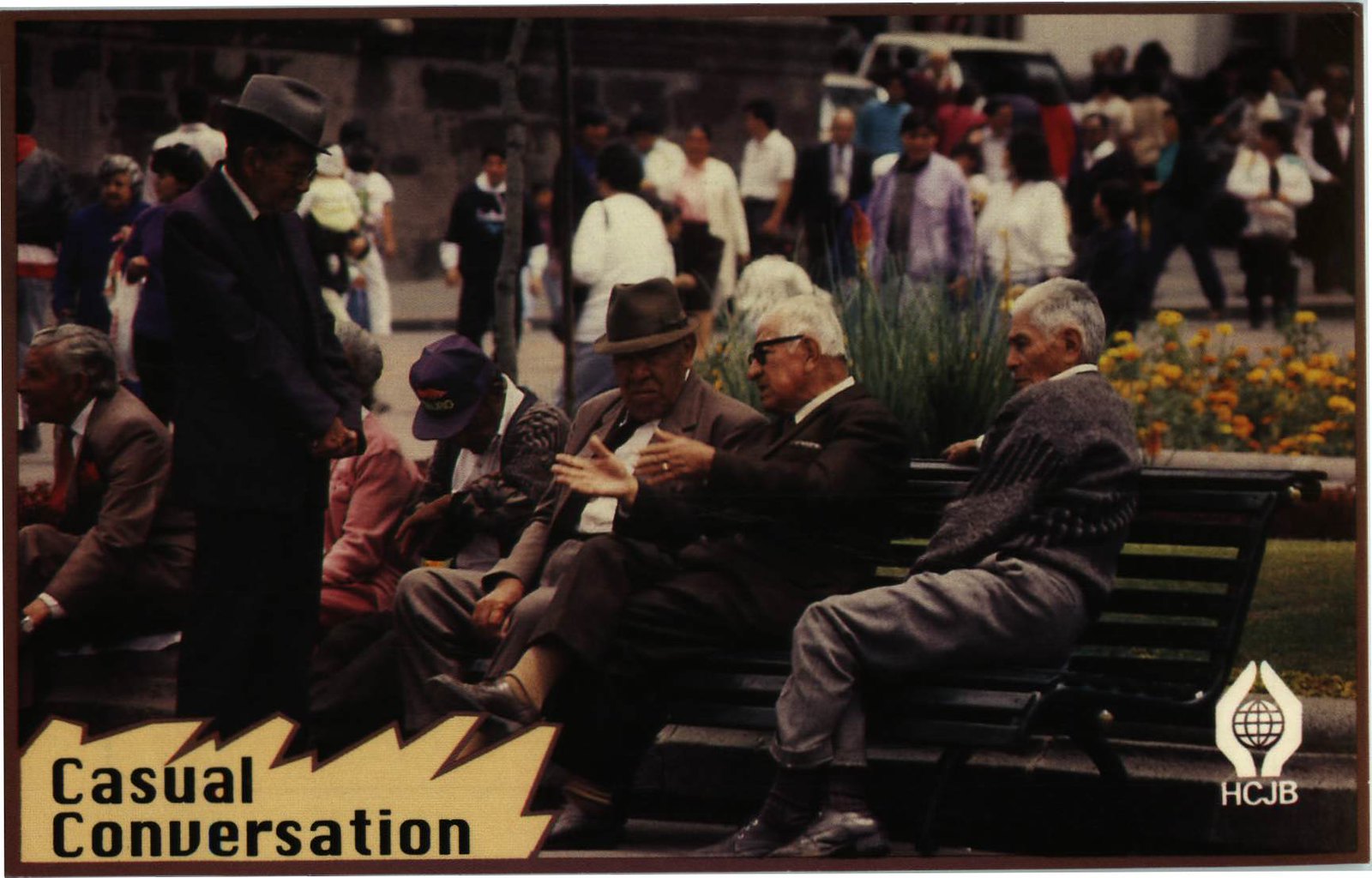In this outdoor scene, three elderly men are seated on a black bench, engaging in an animated discussion. The man in the middle gestures with his hands while the others point to their left, indicating a lively conversation. Adjacent to them on the left stands another man, possibly part of their group, facing them. All the men are dressed in suits, except the one on the far right, who is in a sweater.

In the backdrop, a bustling environment unfolds with numerous people walking around, some seated on another bench to the left, and some simply strolling by. A stone building wall frames the scene behind them alongside a partially visible automobile in the upper right corner of the image.

The photograph is bordered by a narrow brown frame. In the bottom left corner, "Casual Conversation" is inscribed in black letters on a beige background. Additionally, the lower right corner features an emblem of two hands cupping the Earth, with the initials "HCJB" displayed beneath it.